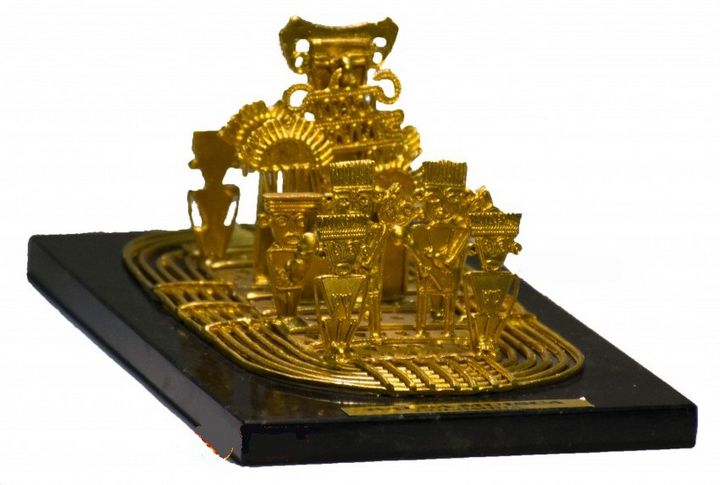This image showcases a striking replica of pre-Columbian gold artwork from Colombia. The piece is displayed on a glossy black square base, around a half-inch thick, which gives it a sleek and sophisticated appearance. The intricately crafted golden artwork on the base features serpentine swirls, spirals, and curves interwoven with small, statue-like figures. These figures, resembling tiki masks adorned with crowns and horns, stand on a golden platform arranged in a circular pattern. The fine details and elaborate designs are highlighted by the luminous gold paint, which contrasts against the dark stand. A gold plate with black writing is affixed to the base, though the text is not legible from the given angle. The entire setup is photographed against a plain white background, ensuring that the focus remains on the intricate and ornate golden artwork.